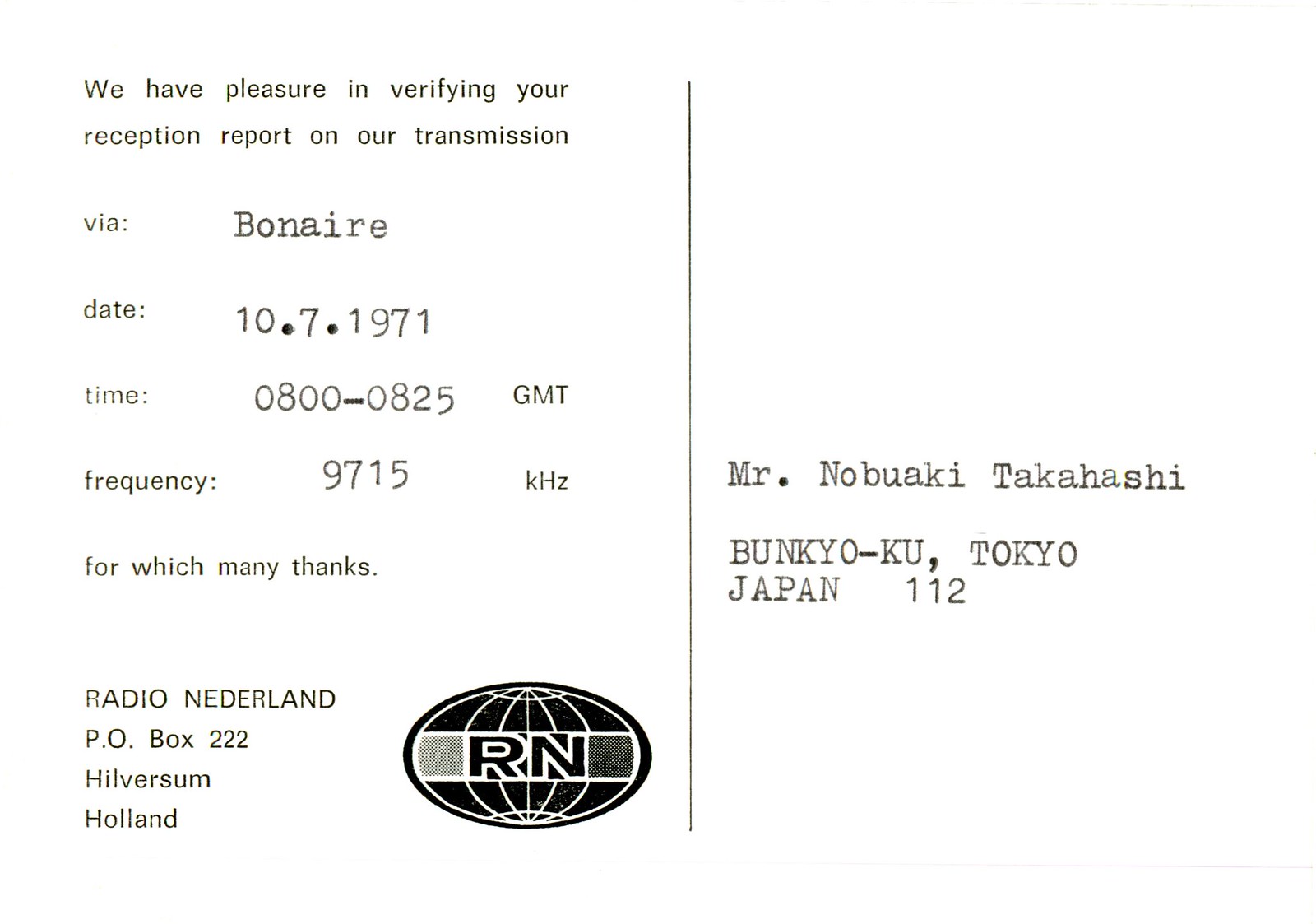The image resembles a scanned postcard with a distinct, dividing black line down the center, giving it a split appearance. The entire background is white, and the left-side features black printed text. At the top, it says: "We have pleasure in verifying your reception report on our transmission." Below this, it indicates the source as "via Bonaire." Further down, it provides specific details: "Date: 10-7-1971," "Time: 0800-0825 GMT," and "Frequency: 9715 kHz," followed by the phrase, "for which many thanks."

At the bottom left, the text reads: "Radio Nederland, P.O. Box 222, Hilversum, Holland." Adjacent to the text is a logo featuring a globe with the letters "RN" prominently displayed. On the right side of the postcard, centrally located, the recipient's name appears: "Mr. Nobuaki Takahashi." Below that, in block capitals, are the address details: "Bunkyo-ku, Tokyo, Japan 112."